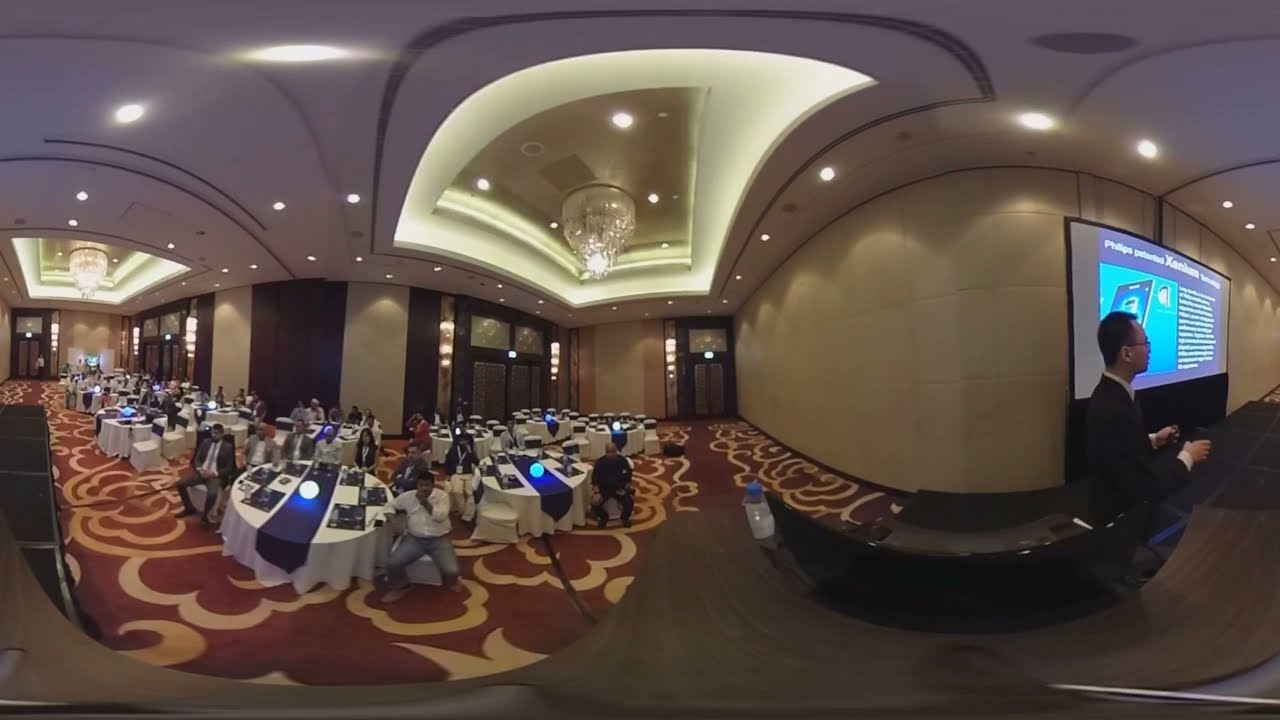The image depicts a large, opulent hotel ballroom or conference hall set up for a formal business dinner. The panorama-style photo reveals a spacious area with elegantly dressed round tables featuring white tablecloths and blue or purple runners, each adorned with a glowing orb at the center. The room's floor has a red and white carpet, while crystal chandeliers hang from the beige and brown ceiling, adding to the luxurious ambiance.

On the left side of the image, numerous people, dressed in black and gray suits and black dresses, are seated around the tables. Their attention is directed towards a stage on the right side of the image. Here, a man in a black suit coat, white shirt, and glasses stands in front of a large whiteboard or projector screen, seemingly about to give a presentation. 

Additionally, there's a photographer in a purple shirt capturing the event from a distance. The overall setting exudes a business-casual atmosphere with a focus on the formal presentation taking place.